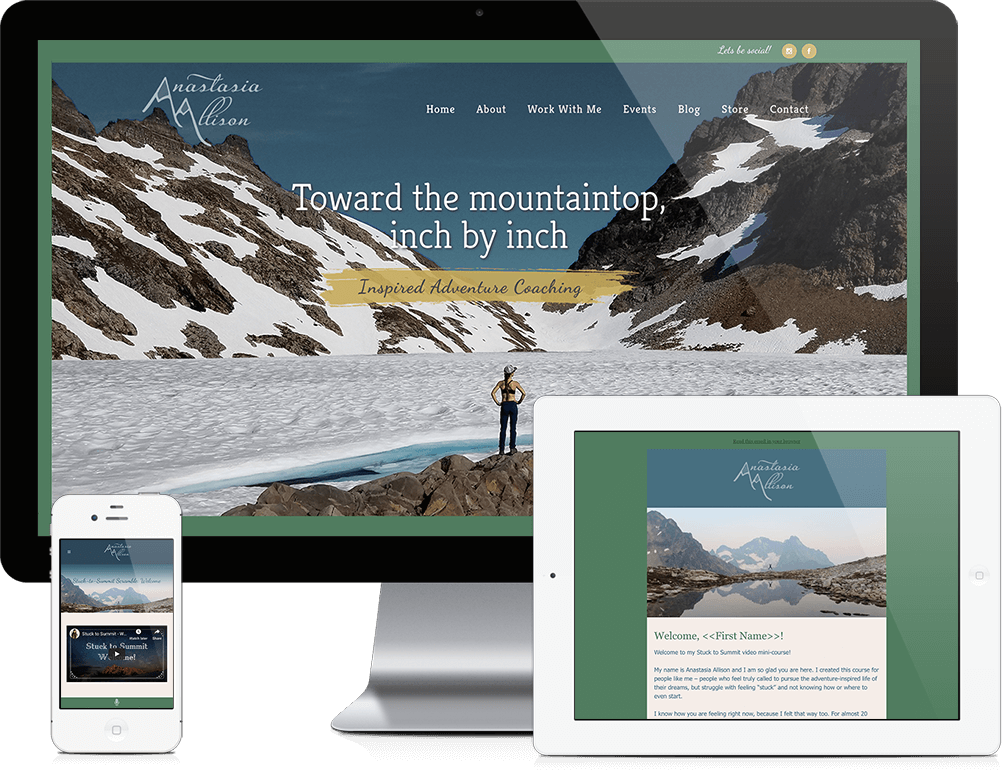The image features a detailed screenshot of a computer monitor with a sleek black border and an inner dark green edge. Displayed on the screen is a breathtaking photograph taken from a high mountaintop vantage point, capturing a rugged, black-and-gray mountain characterized by its jagged peaks blanketed with snow, reminiscent of a glacier. In the foreground, a woman stands confidently in a snowy valley between two imposing peaks. She is dressed in a sports bra, a baseball cap, and tight black leggings, standing on a pile of rocks.

Prominently, the top left corner of the screen displays the name "Anastasia Allison." Below this are menu options: Home, About, Work With Me, Events, Blog, Store, and Contact. Above the woman's image, the motivational text reads, "Toward the Mountaintops, Inch by Inch." An orange banner underneath this tagline highlights the service "Inspired Adventure Coaching." Below this section, the screen is split, showcasing images of modern devices: a white smartphone on the left displaying mountain scenery and a tablet on the right featuring a serene image of a small lake surrounded by mountains.